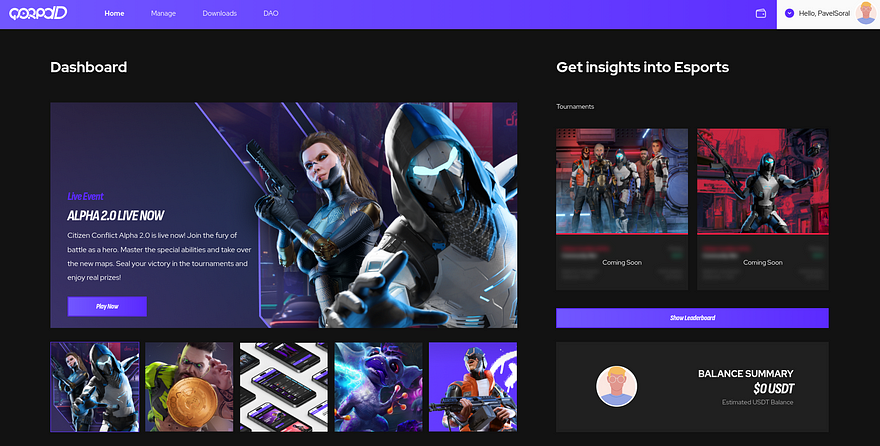This image is a screen capture from a digital platform, featuring a detailed and multi-faceted interface. 

At the top, a royal purple header bar is adorned with white font, displaying the text "Corbid," followed by navigation options: "Home," "Manage," "Downloads," "DAO," and an icon of a wallet. To the right, a greeting in a white box reads "Hello," followed by a username. Adjacent to this is a circular profile icon portraying an animated, blonde-haired character in a blue shirt.

Beneath the header, a dominant graphic proclaims "Alpha 2.0 Live Now" in bold text. The accompanying description heralds the release of "Citizen Conflict Alpha 2.0," inviting users to engage in battle as heroes with special abilities on a new map. Players are encouraged to "Seal your victory in the tournaments and enjoy real prizes." Below this message is a prominent blue button labeled "Play Now." The graphic is adorned with artwork, showcasing three characters: a ponytailed, brown-haired woman with piercing blue eyes and a tattooed arm, wielding a black gun and wearing black gloves with brass and gold accessories; a hooded figure in white armor with a white mask and glowing eyes; and game images like a dark-haired man reaching for a gold coin, simulated cell phones on a white surface, and a purple alien creature with curly purple hair, red eyes, and orange fingers.

On the left side of the screen, in a smaller version of the main graphic, various characters and scenes are displayed. One notable image includes a group of superhero characters standing against a gritty, gray and red industrial backdrop, while another highlights the white-armored, masked figure with blue eyes against a red and black background. Towards the bottom, there are two boxes labeled "Coming Soon."

Further down, a blue box with white text can be seen, followed by a summary section featuring the blonde-haired character in a blue shirt once again. This section details a "Balance Summary" with a balance of "Zero dollars USDT."

Overall, the image showcases a comprehensive and visually engaging user interface filled with characters, graphics, and functional elements.